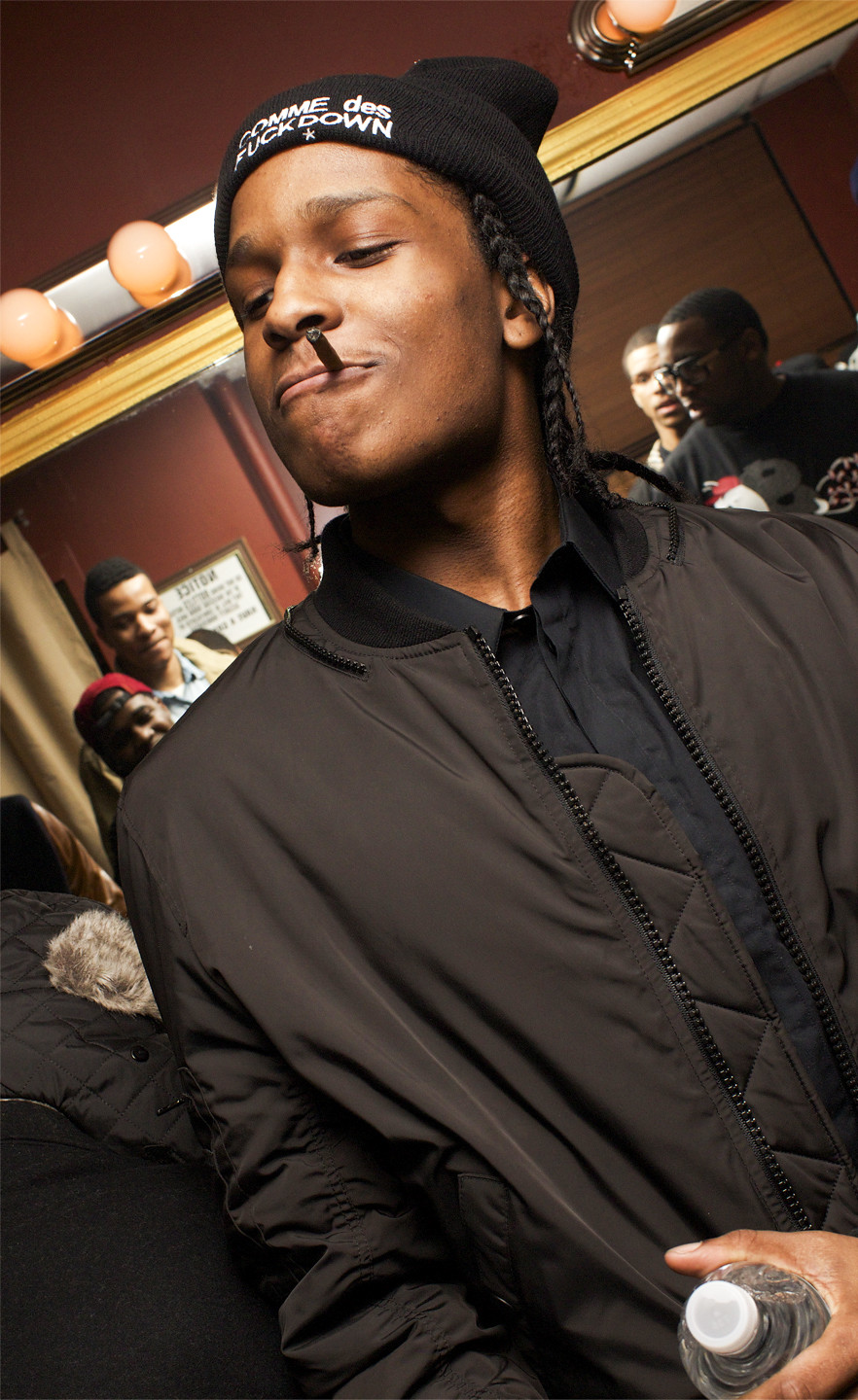The photograph features rapper A$AP Rocky, easily recognizable by his distinctive braids peeking out from under a black stocking cap embroidered with the words "calm the fuck down" in white. He has a blunt hanging from his mouth and a water bottle in his hand, contributing to his nonchalant demeanor. The backdrop appears to be a green room, likely backstage at a concert or performance venue, characterized by its dimly lit, cozy atmosphere. Multiple African American men, possibly his entourage or fellow artists, populate the room. The walls are a mix of dark brown and red, with mirrors bordered by light bulbs, typically used for makeup. Additionally, there is an orange light fixture resembling round balls, adding a soft glow to the scene. A$AP Rocky is wearing a partially unzipped black jacket over a black shirt, with the whole setting exuding a casual, pre-show vibe.